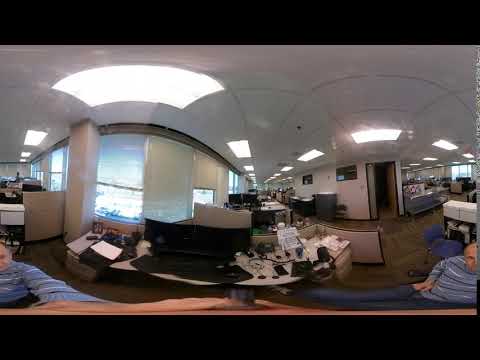In this brightly lit office area, several cubicles are arranged in various formations with white curvature patterns and black trim. The spacious room features numerous embedded lighting fixtures in the white ceiling. Multiple computer desktops and screens dot the area, emphasizing its function as a workspace. 

A man in a blue shirt, a Caucasian male, is prominently seated in an office chair on the right side of the picture, possibly taking the photo with his left hand. Interestingly, there are a couple of other people in the foreground, also in blue shirts with white stripes, adding a uniform appearance to the scene.

The office includes several amenities, such as a bench and coffee makers, enhancing the workspace environment. Windows with partly drawn shades line both the left and right sides, allowing natural light to complement the bright artificial lighting. The image captures doorways and hallways leading to other rooms and areas within the building, contributing to the busy yet organized atmosphere.